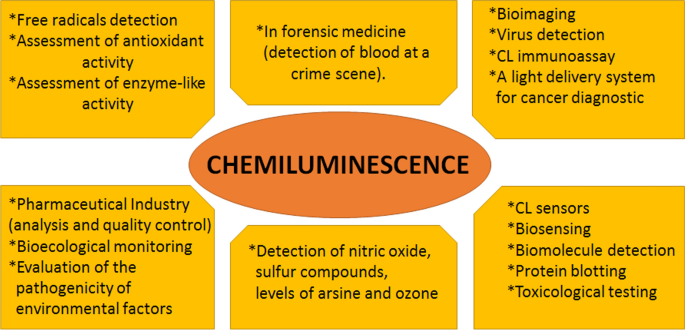The text diagram image features a white background with six yellow rectangles arranged around a central orange elliptical shape. The tops of the rectangles have cut corners. The rectangles are organized with three at the top and three at the bottom, creating a balanced layout. All the shapes contain black text detailing various applications and concepts. The text within the shapes includes phrases such as "free radicals detection," "assessment of antioxidant activity," "assessment of enzyme-like activity," "forensic medicine detection of blood at a crime scene," "bioimaging," "virus detection in the CL immunoassay," "light delivery system for cancer diagnostic," "pharmaceutical industry analysis and quality control," "bioecological monitoring," "evaluation of the pathogenicity of environmental factors," "detection of nitric oxide, sulfur compounds, levels of arsine and ozone," "CL sensors," "biosensing," "biomolecule detection," “protein blotting," and "toxicological testing." The elliptical shape in the center prominently displays the word "chemiluminescence."